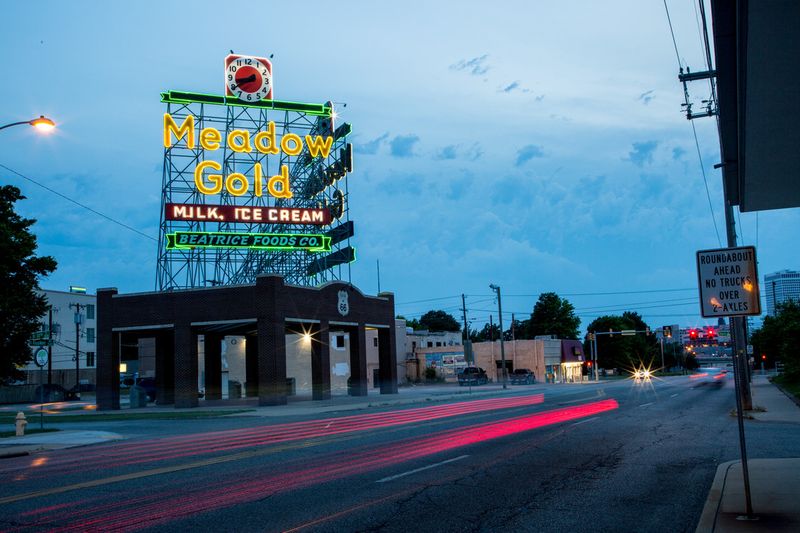This landscape photo captures an urban streetscape at dusk, with a road extending diagonally from the bottom left to the far right corner. Dominating the left side of the scene is a prominent brick building, distinguished by strong, brown pillars. Atop this building, a striking metal structure supports a vibrant neon sign. This sign, a key focal point of the image, features the bright yellow text "Meadow Gold," followed by "Milk" and "Ice Cream" in red, and "Beatrice Foods Co." in green and blue. Above the text, a large red and white clock displays the time as 8:40. The sky hints at approaching nightfall, transitioning from a white to cyan hue near the traffic light. The road itself is marked by streaks of bright pinkish-red light, likely from the long exposure capturing car brake lights. Further into the distance, a traffic light signals red, with blurred headlights visible. On the right side of the street, a small sign on the sidewalk warns, "Roundabout ahead, no trucks over two axles," positioned just under an awning.